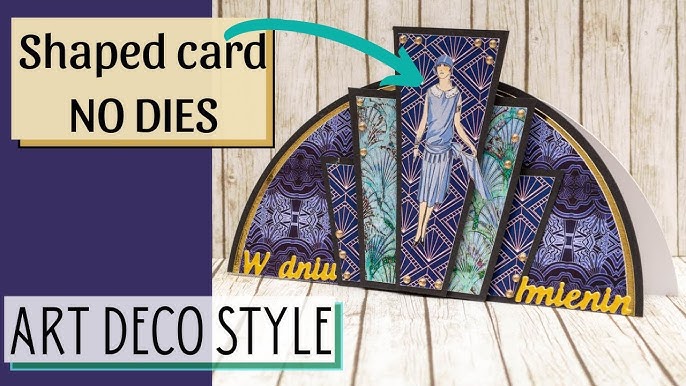**Elegant Art Deco-Inspired Card on a Rustic Background**

The image presents an advertisement for an Art Deco-inspired card, showcased against a rustic wooden backdrop. The overall frame is rectangular. The left quarter is dominated by a rich purple vertical rectangle, while the remainder of the background features white and off-white wooden slats, positioned vertically at the top and horizontally at the bottom, resembling a wall with a shelf protruding.

On the right side of the image, a half-circle card is positioned in an open, standing arrangement. The card's edge is defined by a black outline, followed by a line of gold. The card's background is a deep purple adorned with intricate geometric patterns. Near the bottom, bold yellow text provides additional visual interest.

At the heart of the card, a striking triangular shape, missing its bottom point, displays a captivating blue, red, and white design. A poised woman, dressed in a blue, 1920s-style dress, stands centrally within this triangle. Her figure extends beyond the top of the card, adding an element of dimensionality to the design.

In the upper left corner of the image, a tan rectangle contains black text reading "Shaped Card." Below this, additional text states "No Dies," and a light green-blue arrow directs attention towards the woman in the central design. At the bottom left, a gray rectangle edged in green bears the words "Art Deco Style" in black, emphasizing the card's design inspiration.